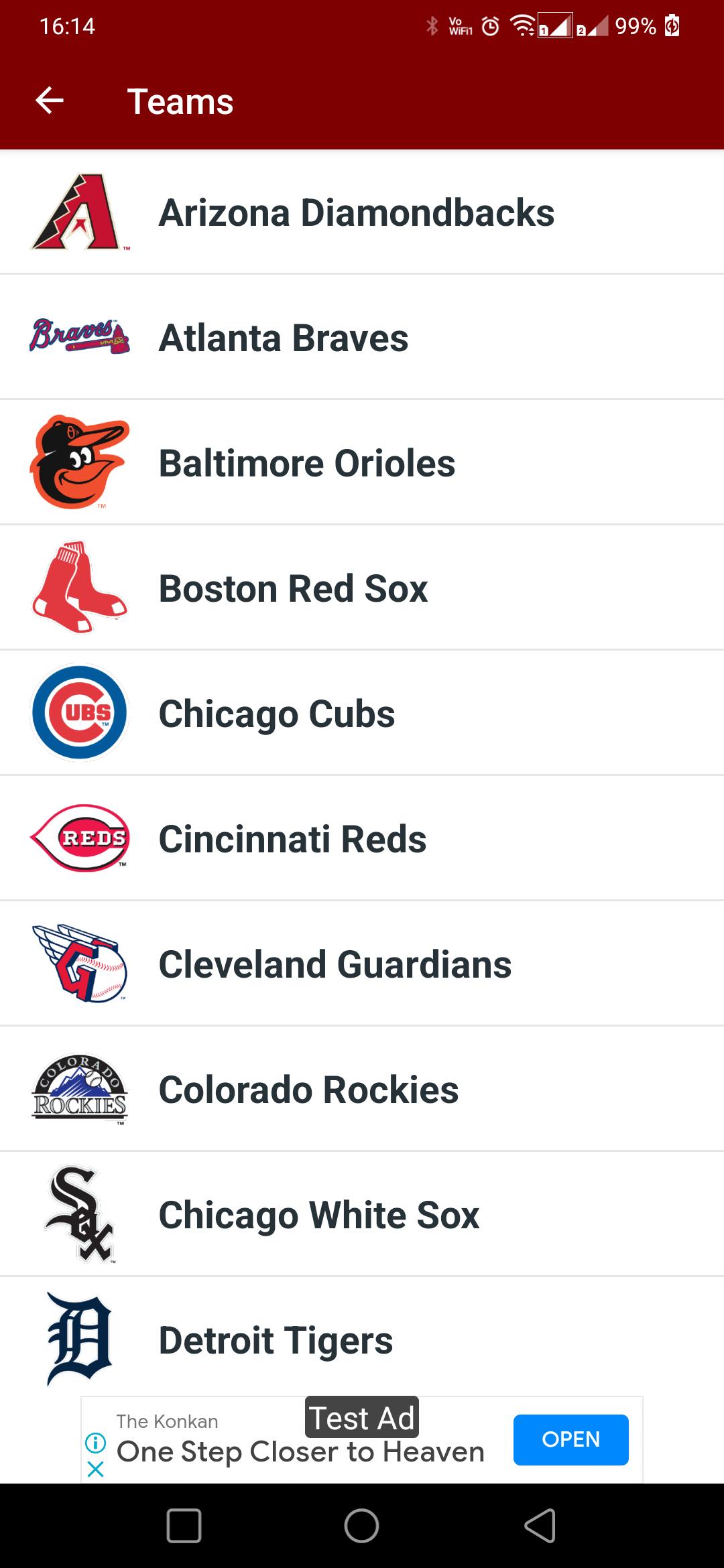The image appears to be a vertical screenshot taken from a mobile device, likely showcasing a sports-related app. At the top of the screen, there's a burgundy text box with a 3D border. Within this text box, standard status indicators are visible, including the time (16:14) on the left, and icons for Wi-Fi, battery (showing 99%), signal bars, and an alarm clock on the right.

Below the text box, the app displays a section labeled "Teams" accompanied by a downward arrow, suggesting it might be a drop-down menu or a collapsible list. The section lists various Major League Baseball (MLB) teams, each represented by their respective logos on the left and names in black font on the right. The names and logos are set against a white background, with each team separated by a gray border. The listed teams include:

1. Arizona Diamondbacks
2. Atlanta Braves
3. Baltimore Orioles
4. Boston Red Sox
5. Chicago Cubs
6. Cincinnati Reds
7. Cleveland Guardians
8. Colorado Rockies
9. Chicago White Sox
10. Detroit Tigers

Further down, there's a banner indicating a test advertisement. At the very bottom of the screen, navigation buttons like "Stop" and "Rewind" are visible, suggesting that this section might be related to media or playback controls within the app.